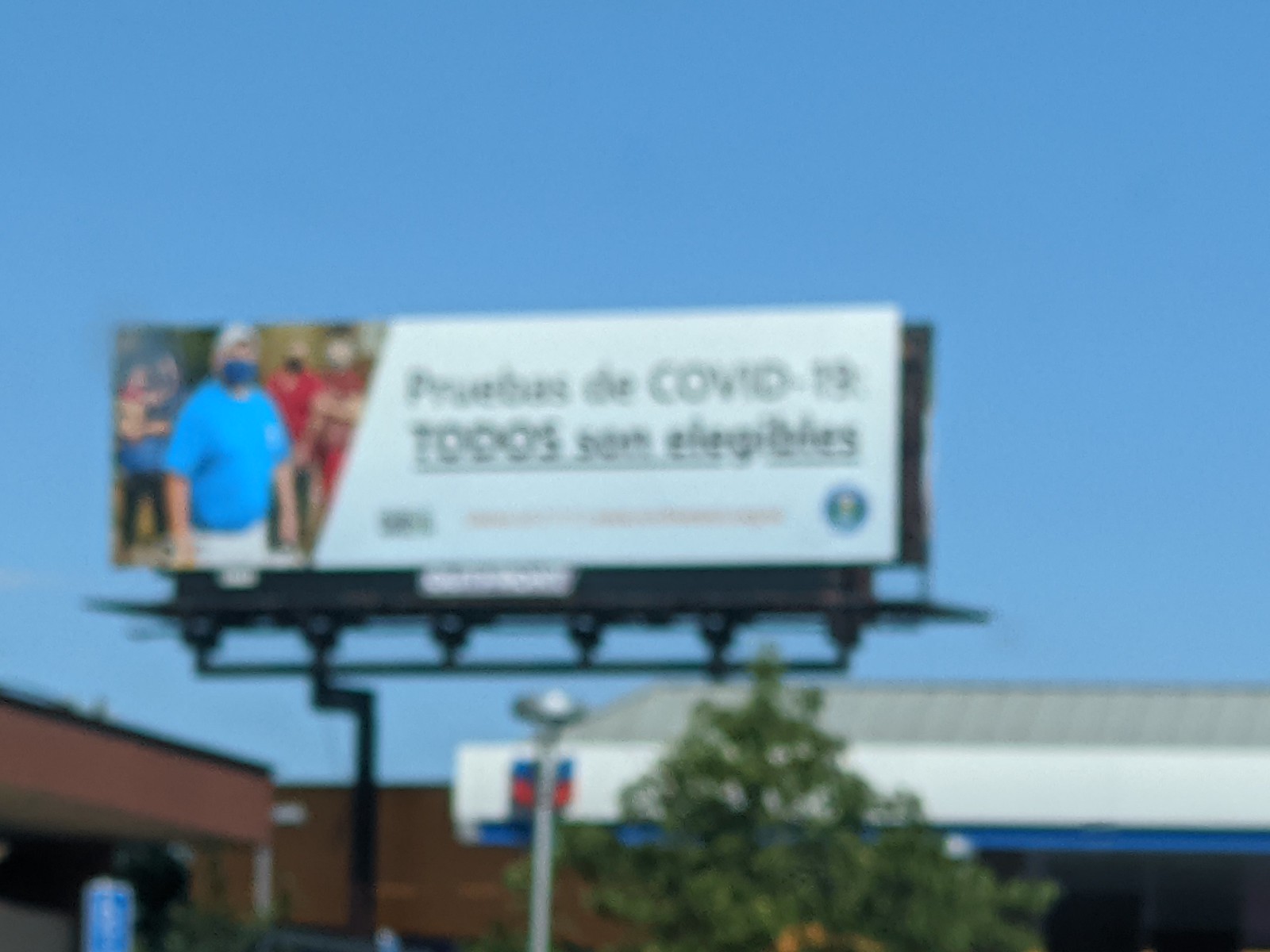This photograph, taken during daytime under a clear blue sky, is notably blurry with a grainy texture, obscuring sharp details. Despite this, certain elements can be discerned. The image captures the tops of two buildings, one featuring a white roof and the other a brown one, along with the upper part of a green tree. A metal structure resembling a street lamp is also visible, alongside a blurry advertisement affixed to a black metal post. The advertisement contains a partially legible photograph of people who appear to be wearing masks, with the only clear text reading "COVID-19."